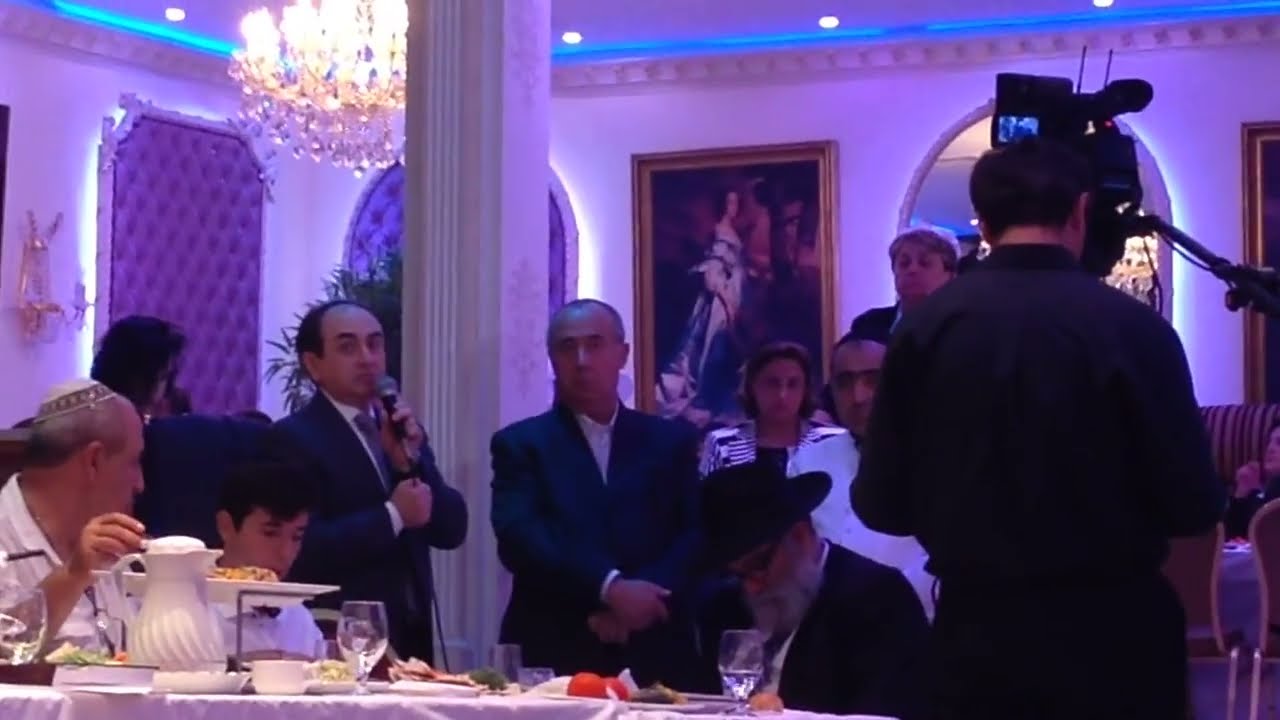The photograph appears to be taken indoors, perhaps in a restaurant, banquet hall, or large conference room, decorated with ornate fixtures, beautiful lighting, and fancy paintings on the walls. The setting suggests an event or celebration with a formal tone, with all men seated at a table in the foreground. They are dressed in suits, with one of them, an elderly gentleman with a white beard, wearing a black suit and hat, and spectacles. Another person appears to be a younger individual. The table is set with goblets, plates of food, and other dishware, although the angle makes it hard to see all the details clearly. One man stands at the head of the table holding a microphone, addressing the group, dressed in a blue suit. Behind him, another man operates a video camera, capturing the event. Adding to the bustling atmosphere, several people in the background are also observing the scene, including a woman and a few others, enhancing the impression of a lively and well-attended gathering. Notably, among the attendees, some men are wearing Jewish yarmulkes, pointing to the possibility of a Jewish celebration. The background is rich with decorated trim and a lit chandelier, adding to the elegant ambiance of the occasion.